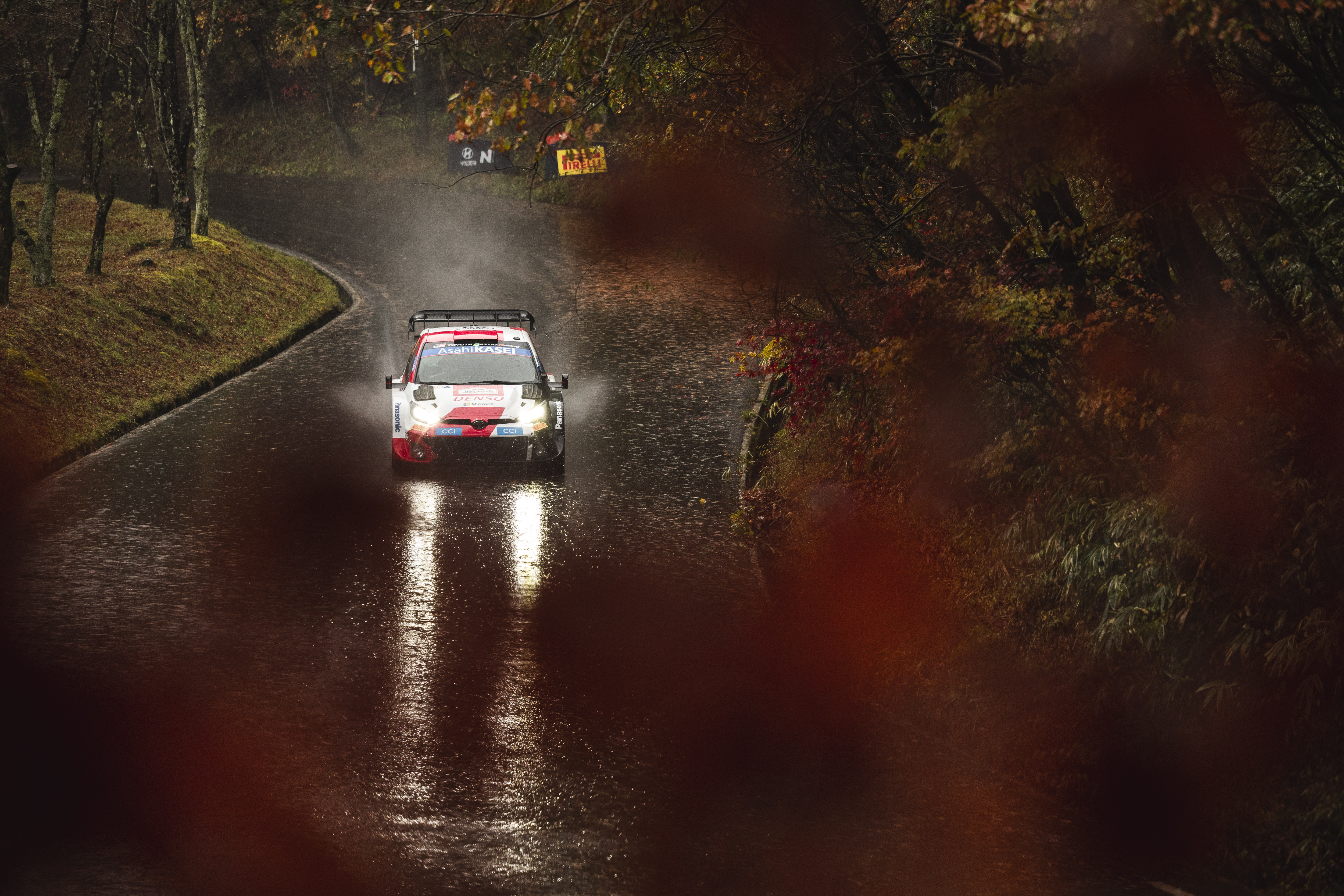The image depicts a nighttime scene of a white racing car driving toward the viewer on a wet, winding road, possibly during a competitive race. Rain creates a damp and reflective surface, causing the car’s headlights to cast a glow on the wet street and mist to rise from the pavement. The car, covered in various advertisements including "DNSO" on the front hood, "CCI" above each light, "ASAHI," and "KASER" on the windshield, has a spoiler across the rear and showcases colors in white, red, and blue. The setting appears forested, with tree trunks and grass visible on the left side of the road and fewer trees on the right. The scene is detailed with blurred red and green hues on the right-hand side of the road. Two signs are visible in the background, one with an ambiguous symbol and "H," and another yellow sign partially reading "I-R-E-E-L-L."